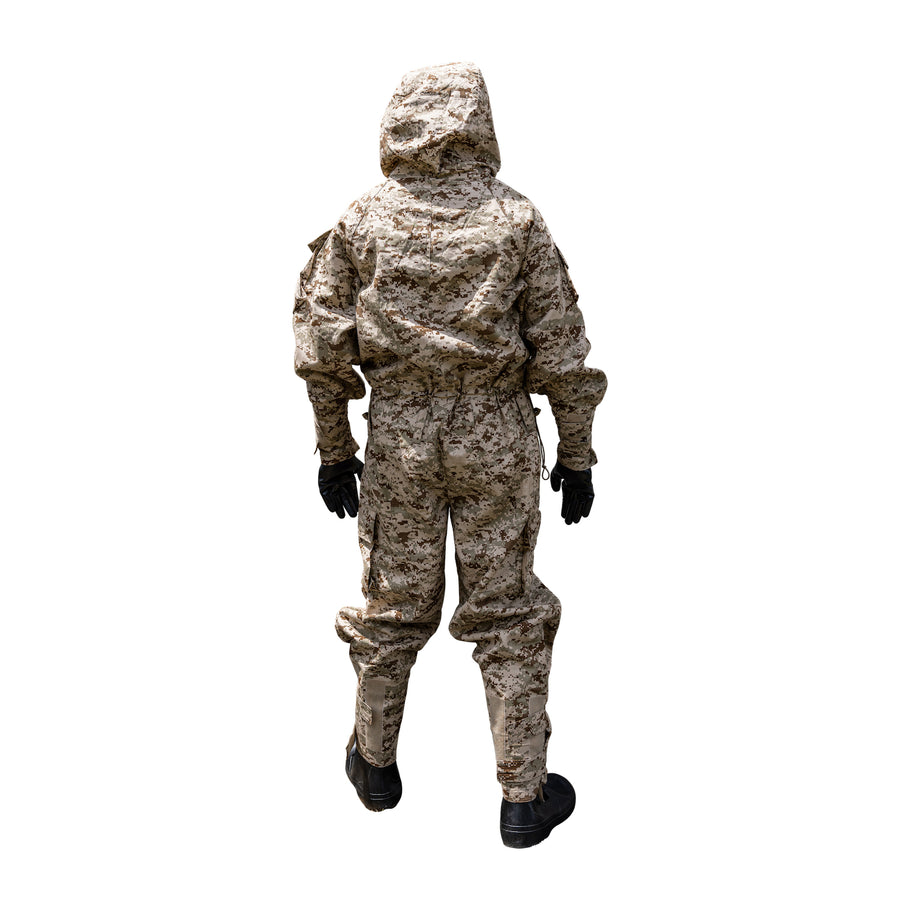This photographic image features a person seen from behind, wearing a full-body, one-piece desert camouflage jumpsuit. The jumpsuit, made from a material resembling Tyvek or a military uniform, is characterized by its cream, light olive, light tan, and brown camo pattern typically seen in hunting gear. It covers the entire body, extending down from the hood to the ends of the wrists and legs, emphasizing a protective, utilitarian design. 

The hood is pulled up over the person’s head, obscuring their identity and adding to the militaristic look. The suit includes long sleeves and is cinched at the waist, providing a tailored fit. The jumpsuit is equipped with multiple functional pockets, notably cargo pockets on the pants' legs and additional pockets on the upper arms. The outfit is completed with black leather gloves and black boots, both contributing to the rugged appearance. The person stands in a neutral position, with feet slightly separated and hands hanging loosely by their sides. The arms are not touching the body, creating a relaxed stance that contrasts with the utilitarian attire.